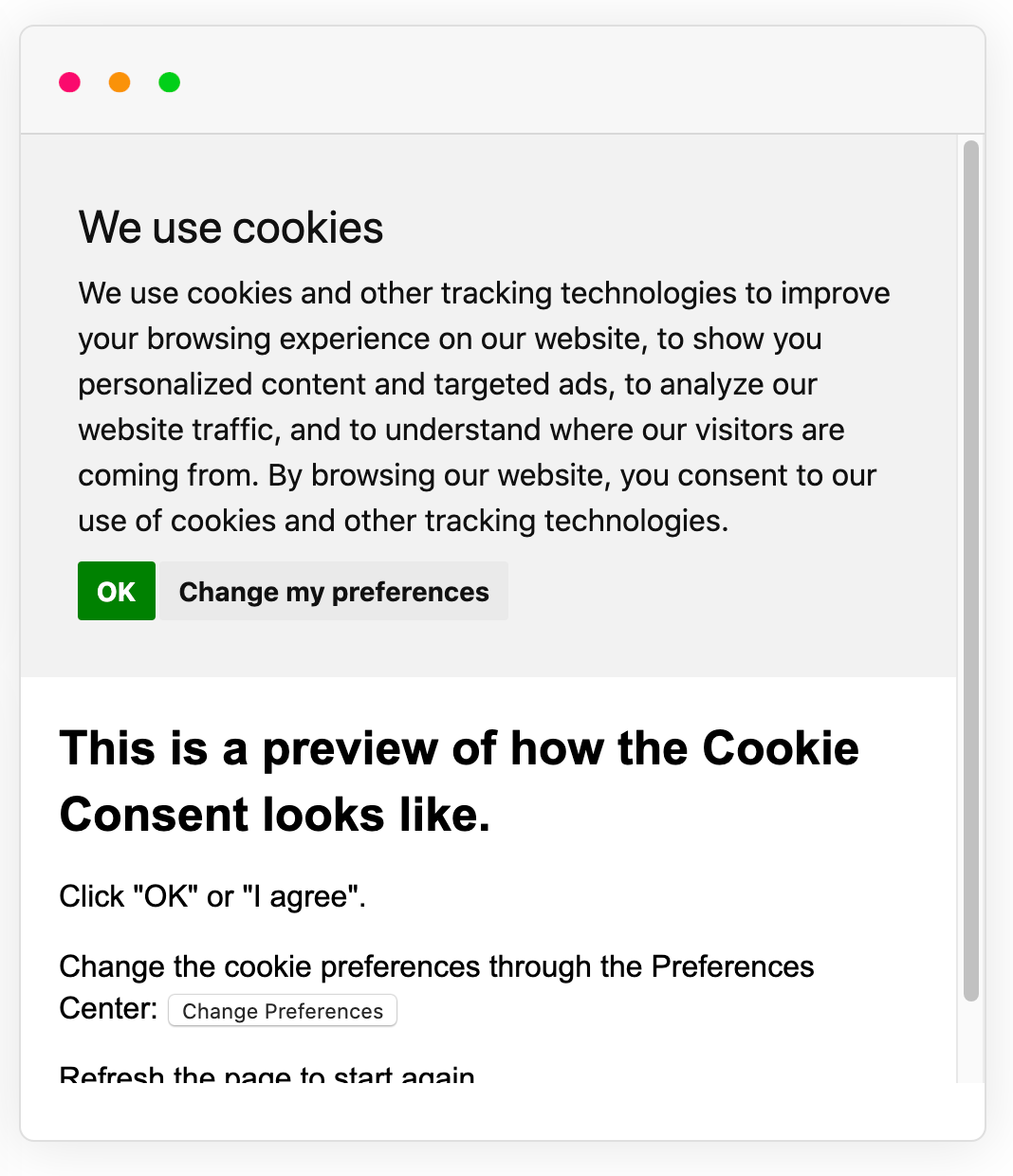The image depicts a cookie notification from a website. At the top of the notification, there are three small dots colored red, orange, and green, resembling the buttons on a browser window. Below these dots, in a light gray area, the text states: "We use cookies and other tracking technologies to improve your browsing experience on our website, to show you personalized content and targeted ads, to analyze our website traffic, and to understand where our visitors are coming from. By browsing our website, you consent to our use of cookies and other tracking technologies."

Further down, there are two buttons: a green box labeled "Okay" and a darker gray rectangle labeled "Change my preferences." Below these buttons, a white box contains additional information: "This is a preview of how the cookie consent looks like. Click okay or I agree. Change the cookie preferences through the preferences center." Another button here says "Change preferences."

At the very bottom of the notification, a phrase partially visible states: "Refresh. Refresh the page to start again." Alongside the entire section on the right side, there is a scroll bar that can be used to navigate the rest of the message, which extends beyond the visible portion of the image.